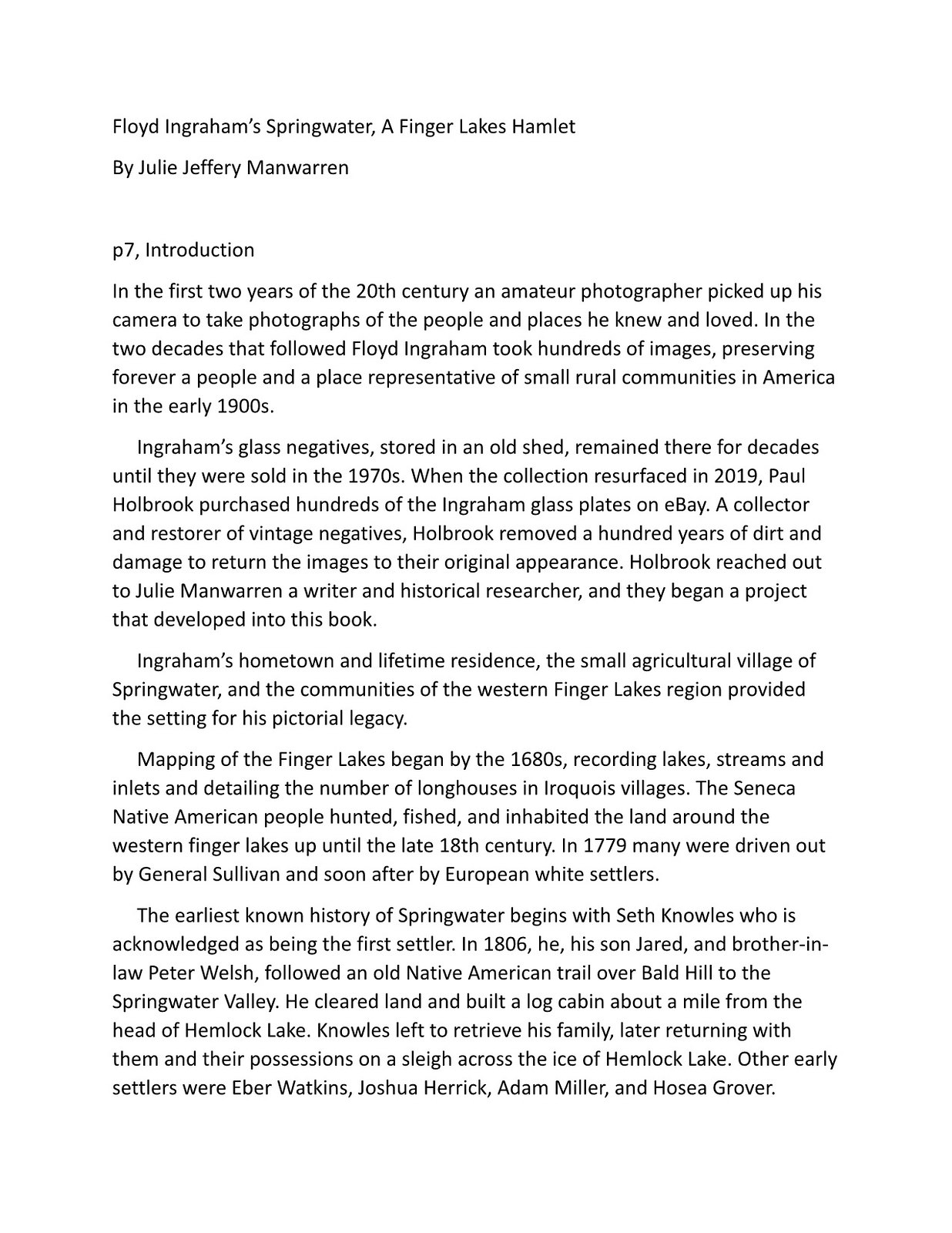This image showcases a printed document on a white background with black text. At the top of the page, it prominently reads "Floyd Ingram's Springwater: A Finger Lakes Hamlet," credited to Julie Jeffrey Mann Warren. This is identified as "Page 7, Introduction." The document consists of five distinct paragraphs, detailing various aspects of the topic. The first paragraph contains five lines, the second paragraph seven lines, the third paragraph three lines, the fourth paragraph five lines, and the fifth paragraph seven lines. The content elaborates on the history and contributions of Floyd Ingram to the hamlet of Springwater, an agricultural village in the Finger Lakes region, with references to historical details dating back to the 1600s.